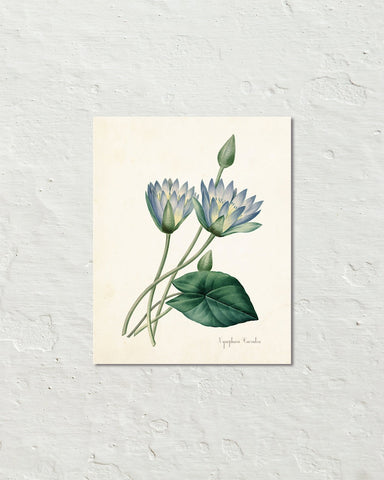A photograph of a vibrant floral illustration hangs against a textured white stucco wall. The photograph, set on an off-white paper with a light yellow background, showcases a detailed portrayal of a plant. In the center, five stems gracefully curve upwards and to the left. The two topmost flowers are in full bloom, boasting petals in shades of blue and purple intermingled with hints of green. Below these, two buds remain closed, resembling teardrops in shape. A large, dark green leaf with prominent veins emerges from the lower section of the plant. On the bottom right corner of the photograph, beneath the leaf, is a small, cursive inscription that possibly indicates the artist's name or the name of the plant, though it is too fine to decipher. The entire piece appears thoughtfully displayed, perhaps intended for artistic appreciation or for showcasing on a website.